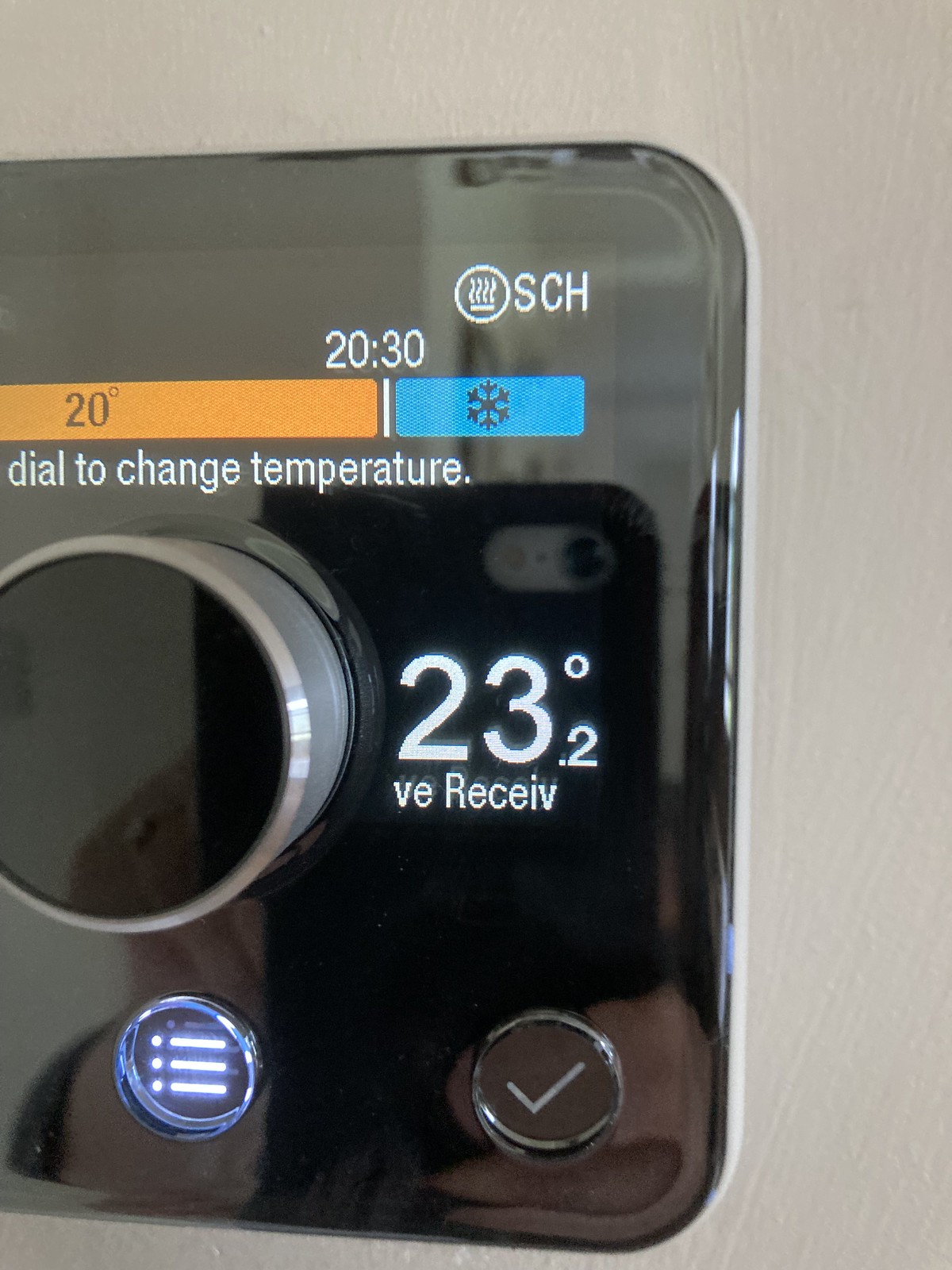The image shows a close-up of a large smartphone screen occupying approximately 80% of the frame. The phone is positioned on the left side of the image and is oriented horizontally. The background is a white, textured wall with several paint splotches, giving it an uneven appearance.

On the phone screen, which is also displayed horizontally, the word "SCH" can be seen prominently along with a circular logo in white. In the center of the image, there is a digital time display showing "20:30". Below this, a temperature reading appears as "20°" encased within an orange rectangular border. To its right, a smaller blue-bordered rectangle contains a black snowflake symbol, indicating a cooling or air conditioning function.

Further down, there is instructional text reading "dial to change temperature" situated above a large circular dial. This dial features a gray outer layer and a black inner core, with "23°" displayed to its right, likely representing the current temperature setting. Below the dial, another small, illuminated circular element with a white light displays a grid pattern comprising three vertical dots intersected by horizontal lines, adding to the intricate details of the interface.